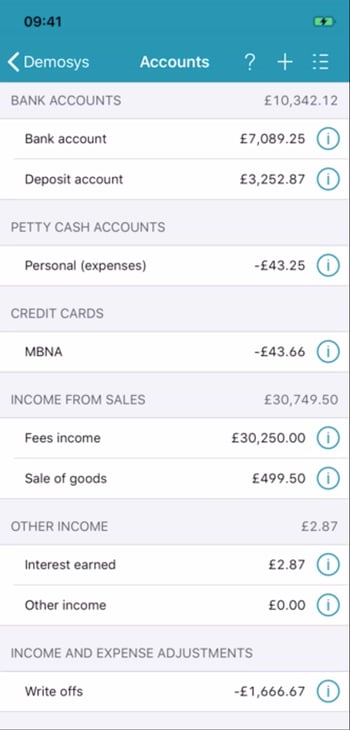Here's a refined and detailed caption based on the provided voice description:

---

This image appears to be a screenshot from a mobile phone interface, showcasing a financial dashboard. At the top of the screen, there's a blue status bar. On the left, it displays the time "9:41" in black. On the right, there's a green battery icon indicating a full charge. In white text, a back arrow is positioned on the left side, followed by the label "Demo," with "Accounts" centered in the middle. Towards the right, there's a question mark icon and an icon with three dots or squiggly lines.

Below the status bar, the main content is displayed on a light grey or white background. The text reads:

- **Bank Accounts**
  - Overall balance: £10,334.12 (GBP)

  - **Bank Account:** £7,089.25 (information icon)
  - **Deposit Account:** £3,252.87 (information icon)

- **Petty Cash Accounts**
  - Personal Expenses: -£43.25

- **Credit Cards**
  - NBNA: -£43.66

- **Income**
  - Income from Sales: £30,749.50
  - Fees Income: £30,250.00
  - Sale of Goods: £499.50
  - Other Income: £2.87
  - Interest Earned: £2.87
  - Other Income: £0.00

- **Income and Expense Adjustments**
  - Write-offs: -£1,666.67

Each entry comes with its own small, round informational icon, providing additional context or details when tapped.